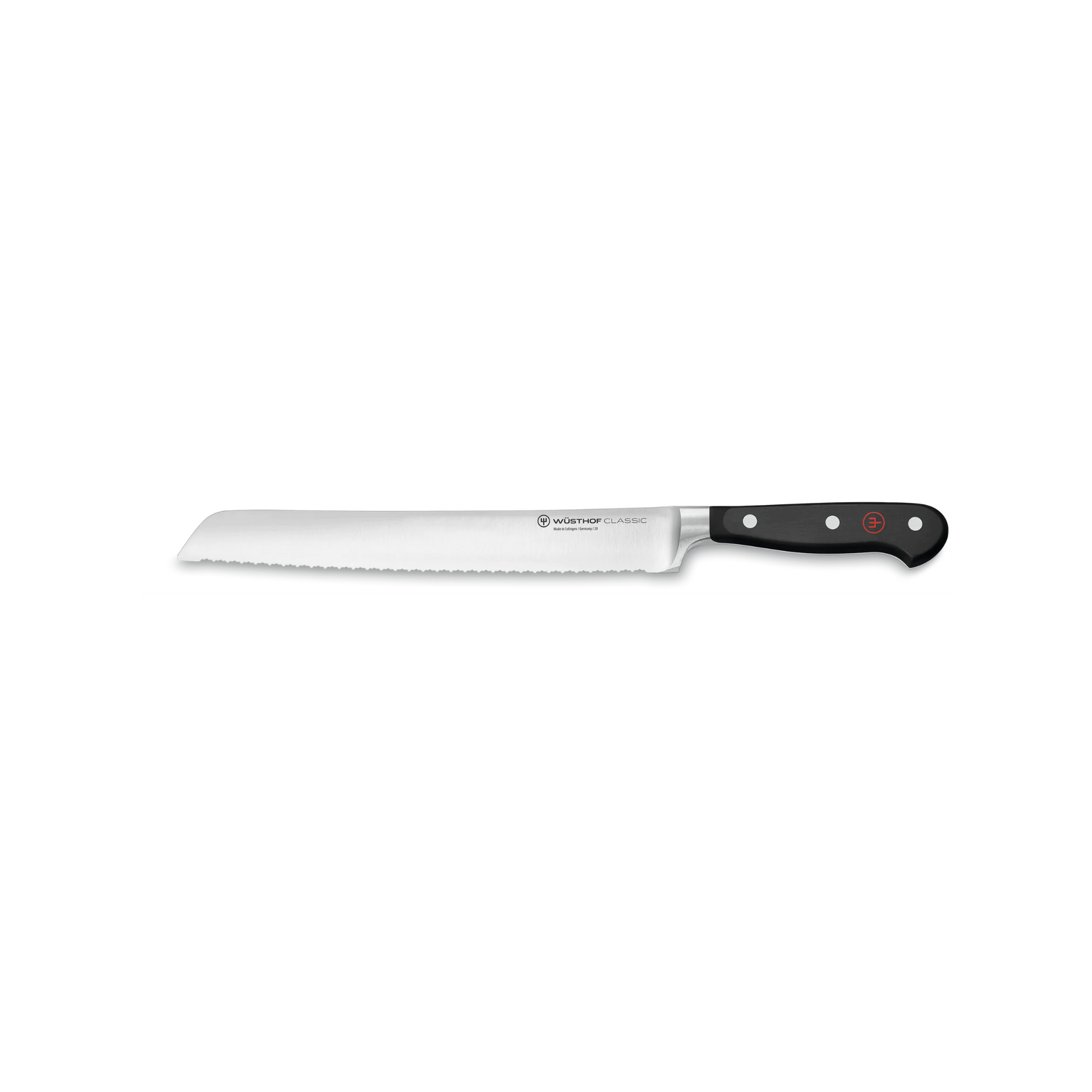This highly detailed photographic image captures a Wüsthof Classic serrated knife set against a stark white background. The knife features a long, polished stainless steel blade, which is approximately three to four times the length of its black handle. The top of the blade is straight with a slight, downward curve near the tip, forming an angle of about 130 degrees. The bottom edge of the blade is serrated, making it ideal for slicing through bread or other similar items. The handle, adorned with three silver fasteners, also sports a distinctive red and black trident logo on the side, with a thin red circle encasing the trident emblem. On the blade itself, near the handle, the text "WÜSTHOF Classic" is prominently displayed, with some smaller, unreadable print beneath it. A similar black trident logo accompanies the text, aligned vertically, contrasting with the red horizontal trident logo on the handle.